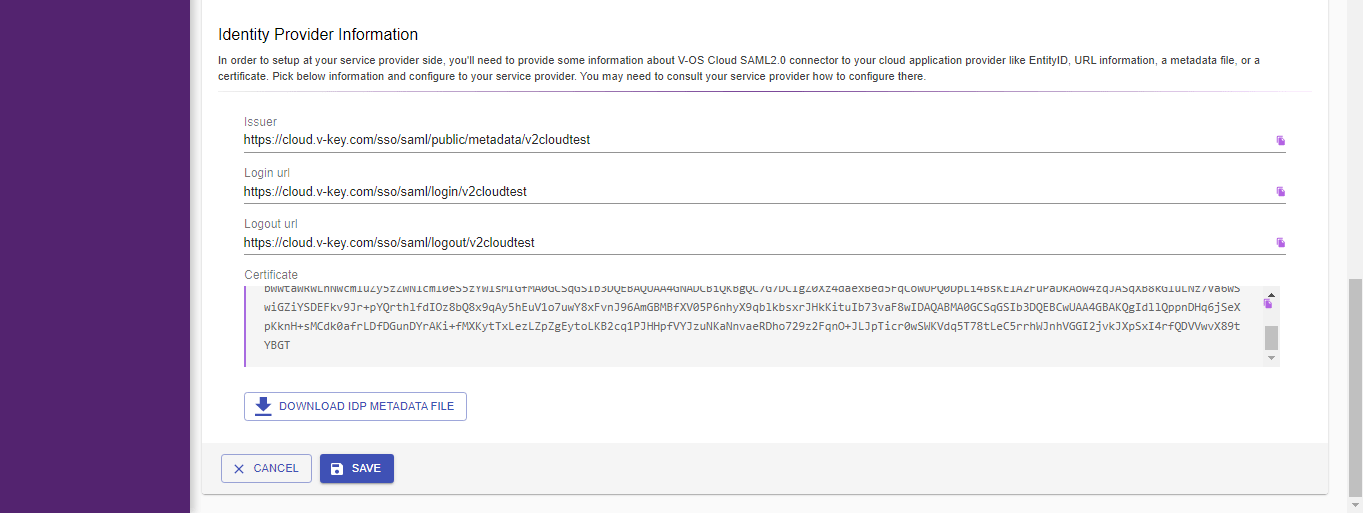A cropped screenshot showcases the identity provider information section of a cloud platform admin panel. The interface features a prominent, thick, purple vertical border along the left edge, contrasting with the white background of the main webpage body. 

At the top, the header "Identity Provider Information" is displayed in bold black text. This is followed by a brief description section, highlighted by a noticeable thick gray horizontal line that serves to demarcate the upper and lower parts of the page.

The detailed interface contains three text boxes designated for inputting login URLs and an issuer key. Below these fields, a certificate section is visible, complete with a scrollbar allowing users to scroll through and read the entire certificate document.

Further down, a white bar with barely legible small text includes an option to download a 15 megabyte metadata file. At the bottom of the interface, two actionable boxes are prominently displayed on the left side: a blue-outlined "Cancel" button and a purple "Save" button, encouraging user interaction.